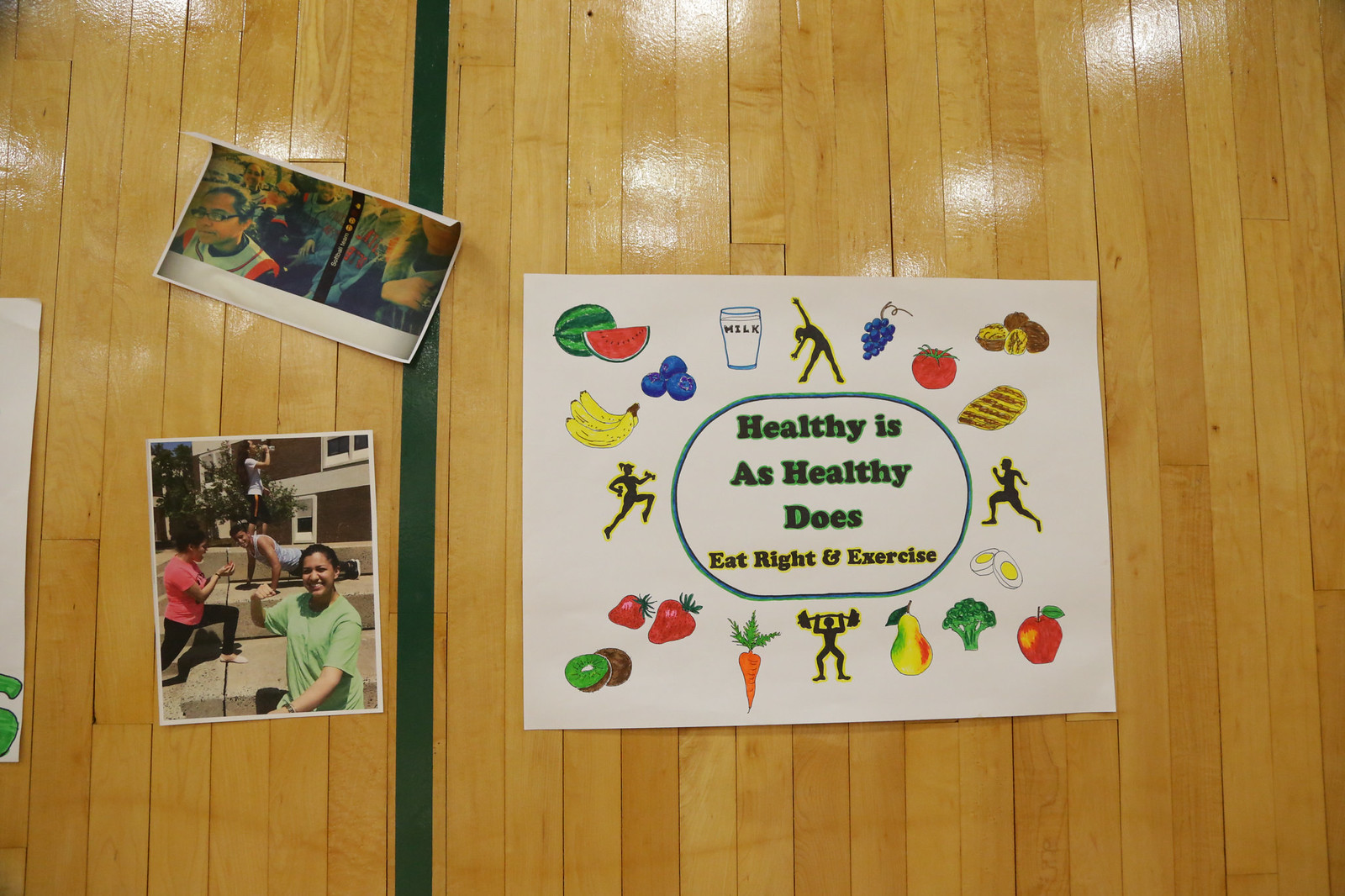This photograph captures an arrangement of multiple printouts spread out on a glossy, wooden floor resembling a gymnasium's surface, complete with visible wood slats and a faint green basketball court line. On the right side, a large white piece of paper is adorned with clip art of various fruits such as watermelon, strawberries, kiwis, bananas, mangoes, broccoli, and apples, alongside illustrations of healthy foods like bread, eggs, and meat. Black silhouettes depict activities such as weightlifting, running, and stretching. Centered in this collage is the motivational text: "Healthy is as healthy does. Eat right and exercise."

To the left, there are two photos printed on paper. The top photo is slightly curled, obscuring the details, but the bottom one clearly shows a group of women who are exercising and smiling at the camera. Additionally, there's a depiction of three people engaged in physical activities: a man performing step push-ups, a woman flexing her arm muscles, and another woman doing stair-stepping exercises. The overall scene promotes a healthy lifestyle through balanced diet and regular exercise.